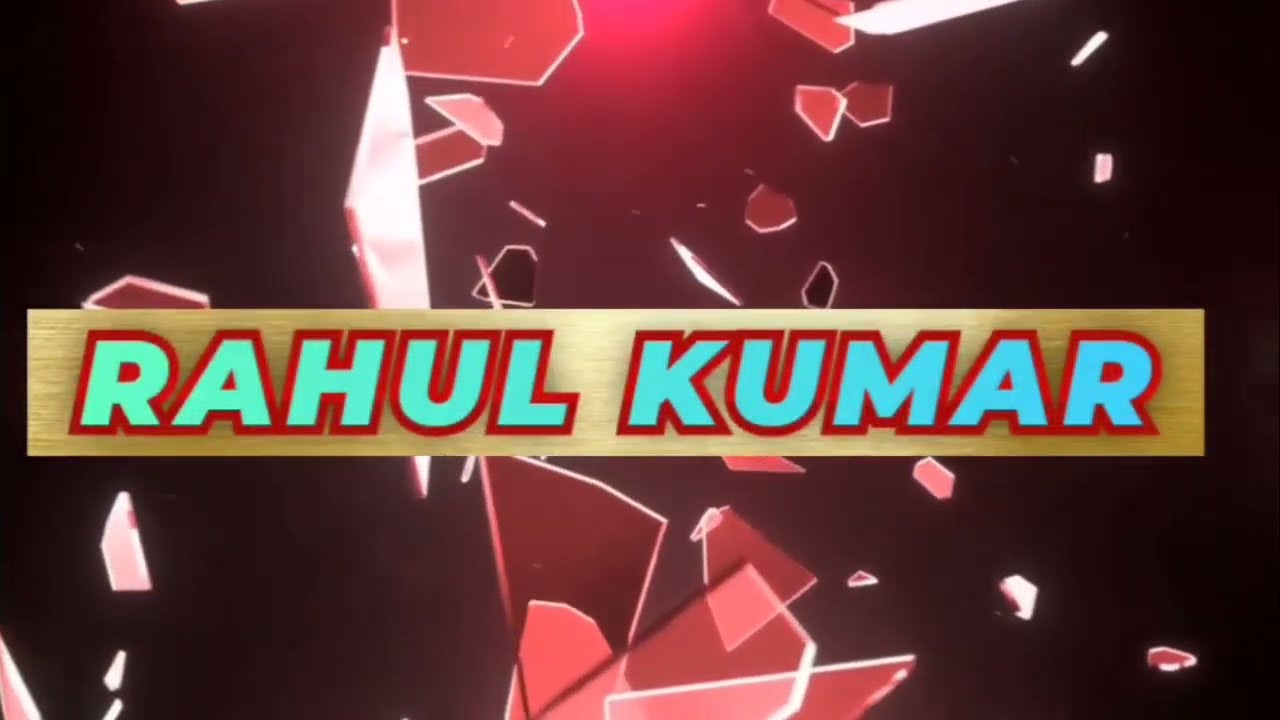This is an introductory graphic, likely a credit for a video. The image features a horizontal rectangular format with a complex 3D rendered background. The background begins with a dark black on the left and right edges, transitioning to a deep red at the center. Glass-like shards, depicted in varying shades of dark red, appear to be in mid-shatter, dispersing across the image. Some shards are suspended in the black sections as well, adding to the dynamic, animated effect. 

The central focal point of the graphic is a gold rectangular bar that spans horizontally across the image. On this bar, the name "Rahul Kumar" is prominently displayed. The name transitions in color: 'Rahul' starts off as a teal green on the left, and 'Kumar' shifts into a light blue on the right, with both names outlined in a vivid red border. Above the graphic, a subtle red light casts a faint glow, adding depth to the shattered glass effect in the maroon-black background.